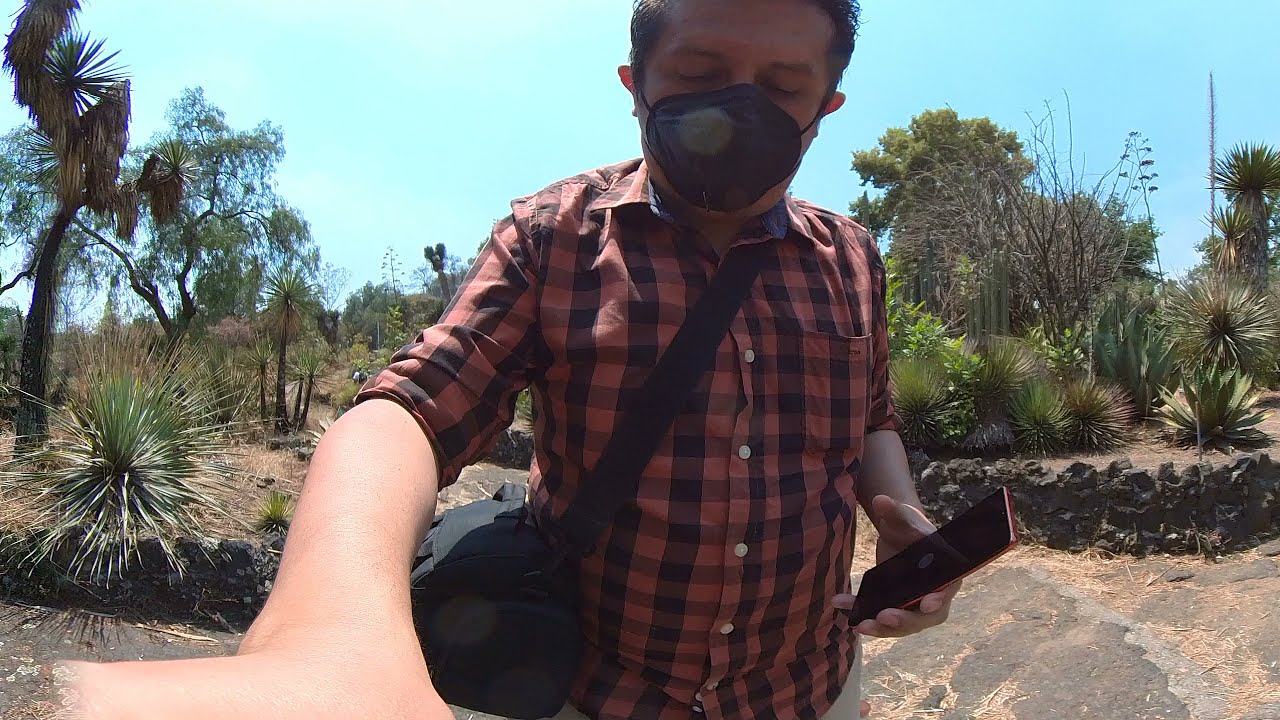The image captures a close-up of a man with short, dark hair, standing in what appears to be a well-maintained public garden characterized by arid climate vegetation. He is reaching towards the camera with his right hand while holding a red cell phone in his left hand. The man is dressed in a red and black checkered button-up collared shirt with the sleeves rolled up and a black crossbody bag slung over his left shoulder. He wears a black face mask and his eyes are closed at the moment of the photograph. Behind him, the backdrop features a variety of desert plants, including cactus, yucca, and palm trees. The ground is light tan and sandy, interspersed with stones, and there is a small, three-foot-tall gray stone retaining wall adding to the picturesque setting. The scene is complete with clear blue skies, adding a bright and open atmosphere to the image.